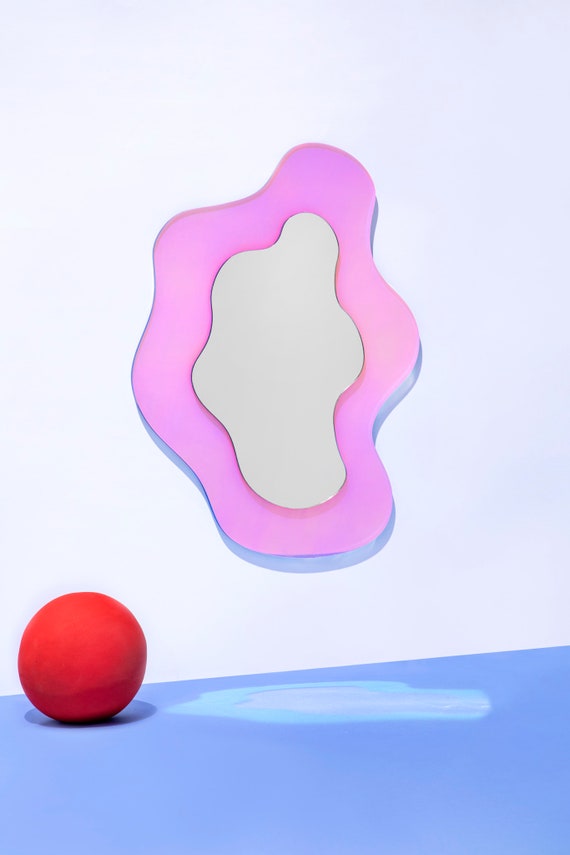The image appears to be an abstract art piece with several distinctive elements. Set against a blank white wall, a squiggly pink object, likely made of a gooey substance, hangs prominently. This pink object encloses a white or potentially mirror-like center, reflecting light and adding depth to the composition. Below, the floor is painted a light blue or periwinkle shade and features a reflective puddle shaped similarly to the squiggly pink object on the wall. This puddle is bluish on the edges with a silvery grey or white center, mimicking the design above. To the left of this puddle, a solid red ball rests on the floor, casting a shadow, and reinforcing the vibrant color scheme. The overall setup is designed to create a harmonious yet intriguing visual balance between the objects and their reflections.